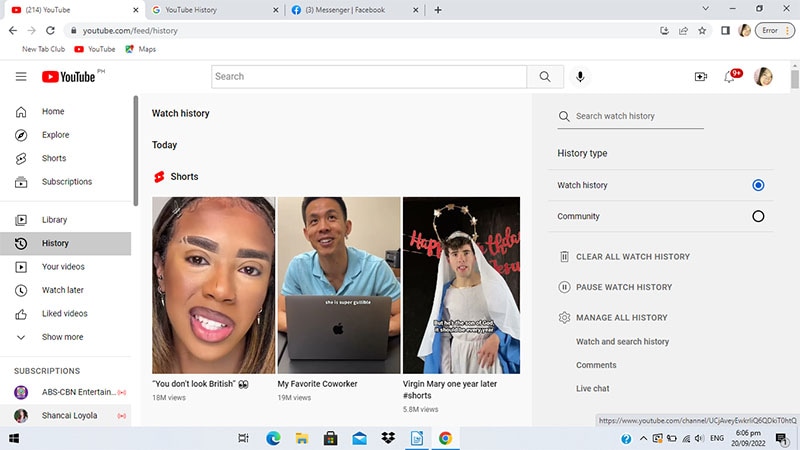The screenshot showcases three YouTube Shorts selections under the user's watch history, each with a substantial view count indicated. The Shorts, characterized by their brief duration, capture varied and engaging content.

1. **“You Don’t Look British”**: Positioned on the left, this Short features an individual with painted eyebrows, slightly smirking at the camera. This intriguing expression adds a playful touch to the video.
   
2. **“My Favorite Coworker”**: The middle Short presents a person smiling warmly while seated behind an Apple laptop. The beige backdrop complements the focus on the individual, creating a cozy and relatable scene.

3. **“Virgin Mary, One Year Later”**: The right-most Short depicts a person dressed as the Virgin Mary, complete with a homemade halo of stars, a head shawl, and a loose garment. The individual, who appears to be male, stands in front of a background adorned with a "Happy Birthday" sign, adding an element of celebration and creativity to the portrayal.

Notably, each of these Shorts has garnered significant attention, with view counts of 18 million, 19 million, and 5.8 million, respectively. The screenshot highlights these popular selections in the user's YouTube Shorts watch history.